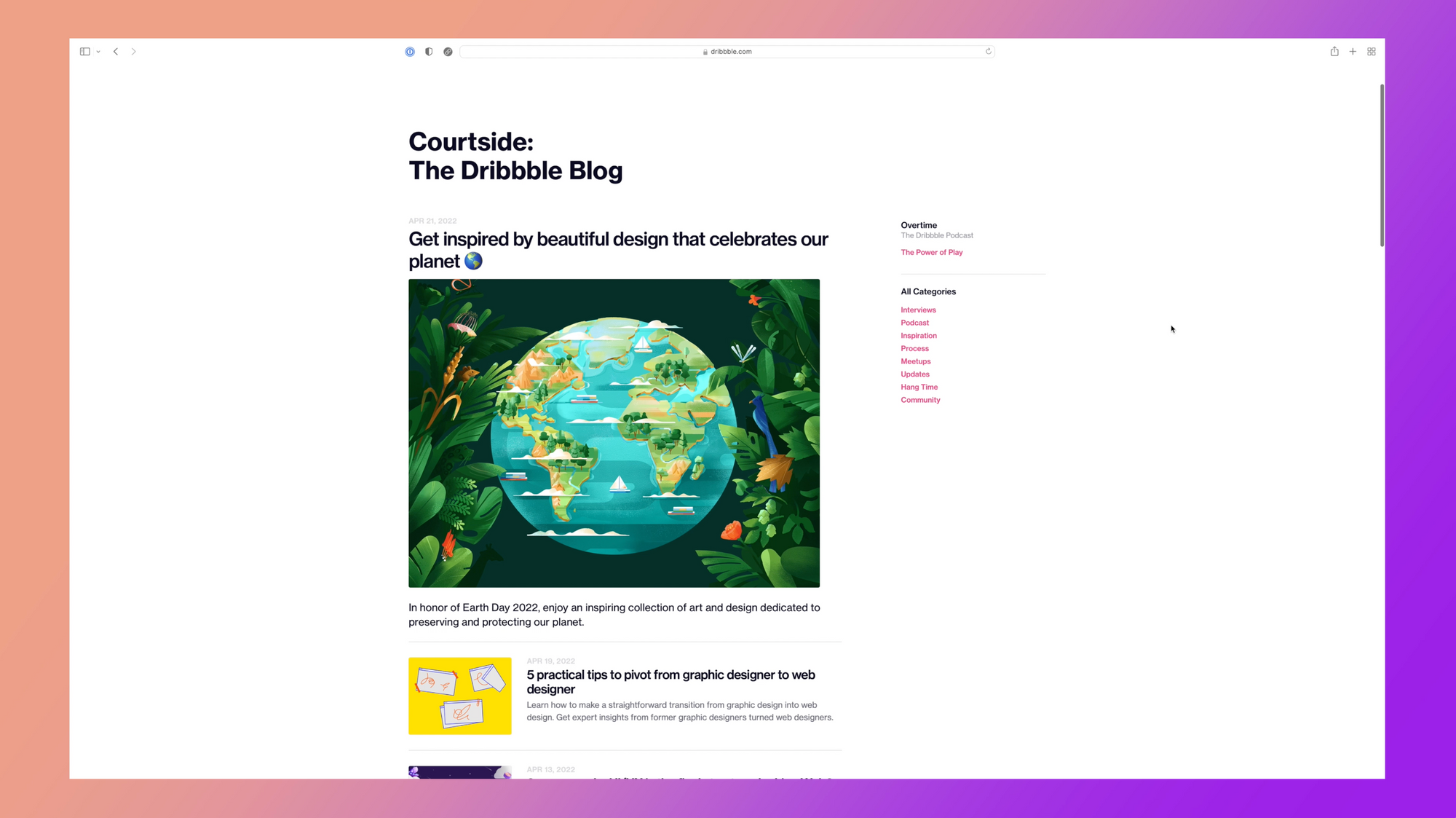A cropped screenshot of a webpage is overlaid on a gradient background, transitioning from pink on the left to light and dark purple on the right. The webpage itself has a white background. At the top of the image is an address bar with very small black text centered within it. Below this, prominently displayed, is the title "Courtside: The Dribble Blog." 

The main feature of the webpage is an article headline that reads, "Get inspired by beautiful design that celebrates our planet." Under the headline is a large thumbnail image depicting a tapestry of Earth surrounded by various plants, with clusters of trees positioned over different continents. 

Beneath this visual, there is a brief description of the article. A thin divider line separates this from the next section, which contains a very small, square thumbnail to the left, accompanied by a title and a short description to the right. The top portion of yet another thumbnail, partially cropped out, can be seen further down the page.